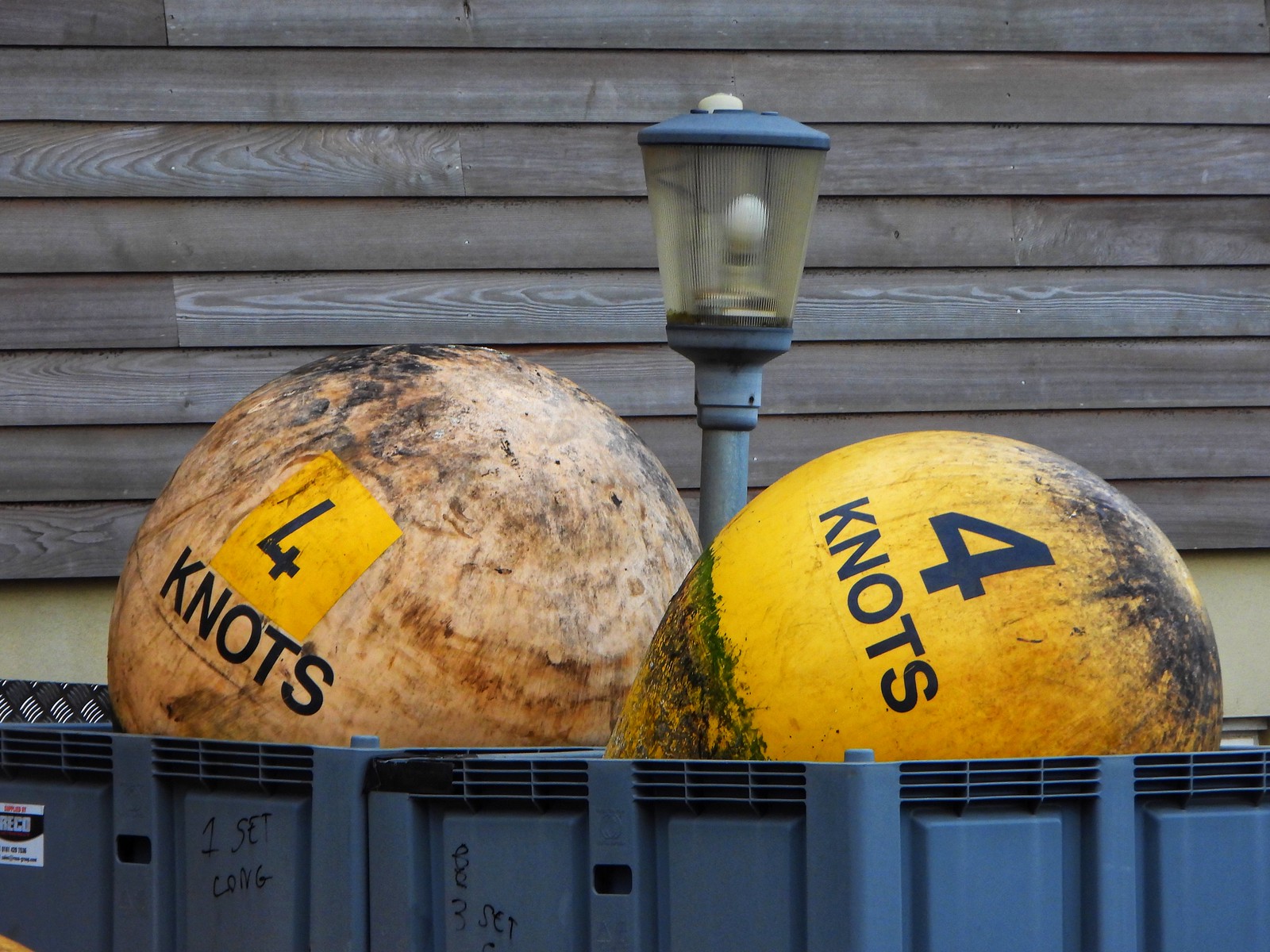In this detailed outdoor image, the backdrop features a dark gray, wood-paneled wall typical of a house, with off-white, yellowish siding beneath it. Central to the composition is an older lamp post with a gray pole and a rounded top with a glass-like cover containing a light bulb. Prominently displayed in front of the lamp are two large, spherical, weathered buoys, suggesting maritime navigation tools marked with the speed "four knots." The buoy on the left is beige with dark smudges, a yellow patch, and the black number "4" followed by the word "knots." The adjacent buoy is orange with black markings and similarly labeled. These buoys rest in a blue plastic bin, possibly Rubbermaid, that features multiple vertical lines and columns. Along the side of the bin in black marker are inscriptions: "one set C-O-N-G" and "three set" in separate columns.